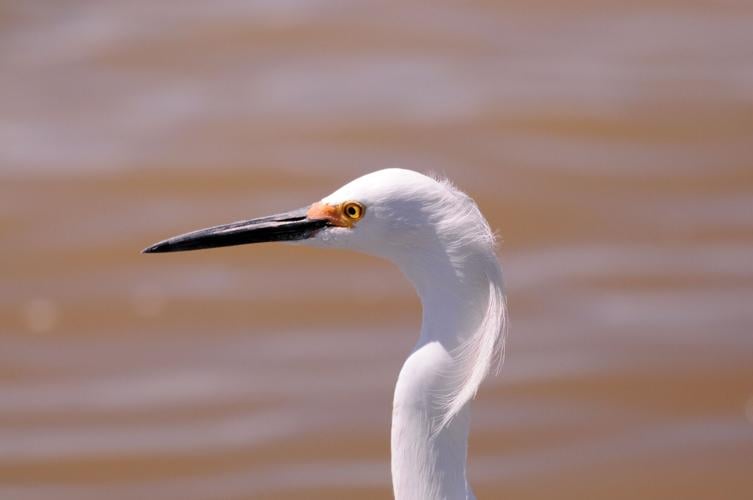This striking wildlife photograph captures a close-up of a bird, presumably a crane or heron, from its neck up. The bird's elongated, slender neck and bright white plumage dominate the composition, drawing the viewer's eye to its intricate details. Its neck, reminiscent of a swan but notably thinner, extends gracefully, occupying about one-third of the image.

The bird sports a unique crest on the back of its head, reminiscent of a 'duck's ass' haircut or a mullet, with a tuft of white feathers that almost resemble horse hair, swept back in a style that could humorously be likened to a 'Donald Trump' look. Its piercing yellow eye, stark against the whiteness of its feathers, adds a sharp contrast, alongside the spongy red skin near its beak, which is characteristic of certain bird species. The beak itself is long and black, perfectly adapted for fishing or pecking at food.

The background is artfully blurred into an abstract pattern of orange, brown, and white streaks, possibly reminiscent of a desert landscape, which makes the bird stand out prominently in the frame. The bird gazes leftward, providing a side profile that emphasizes its striking features and elegant posture. This detailed and captivating image beautifully showcases the bird's distinctive physical attributes against a soft, contrasting background.